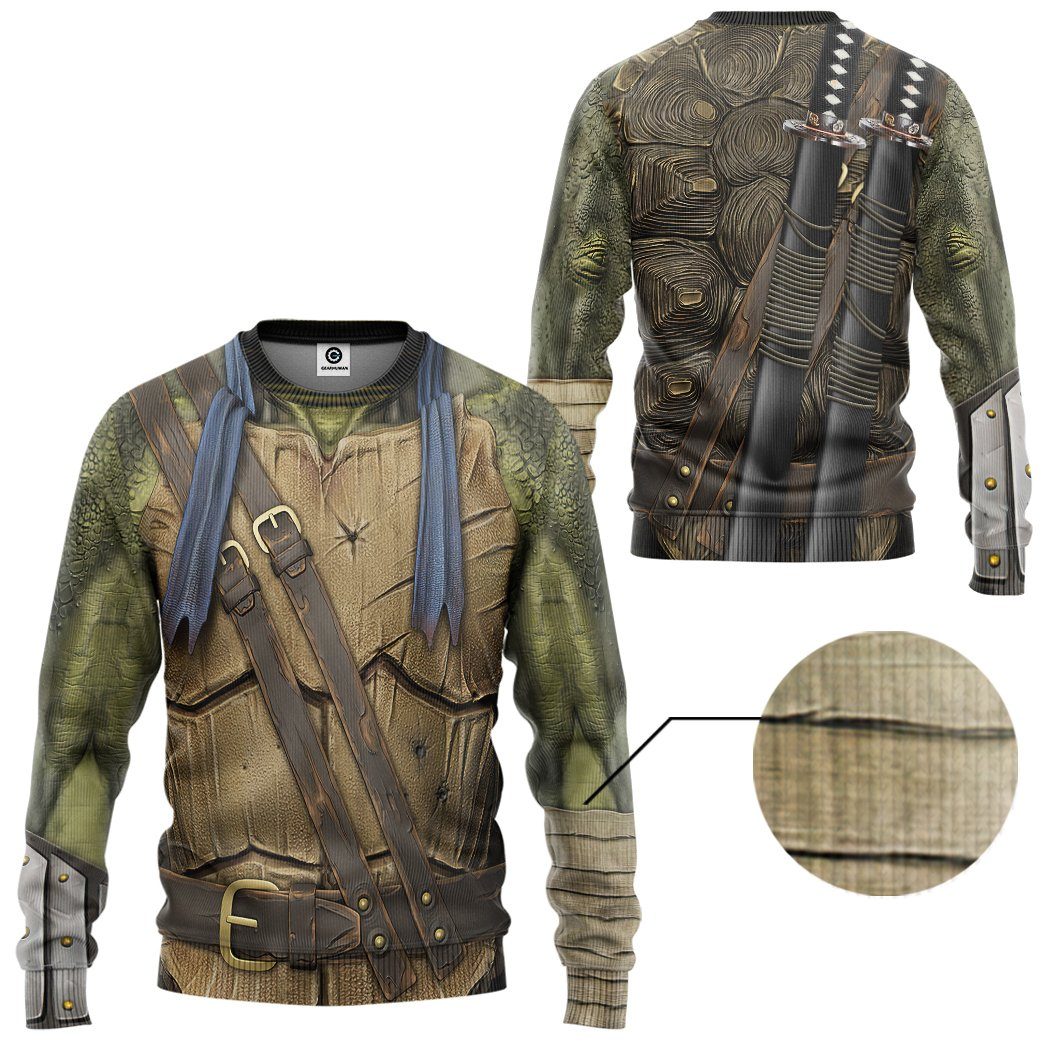This image showcases a detailed Teenage Mutant Ninja Turtle costume shirt displayed against a white background, typical for an online marketplace. The long-sleeve shirt features intricate printing that mimics a warrior's outfit. The front of the shirt depicts leather straps running from the right shoulder to the left hip and a leather belt with a metal buckle at the waist. The arms are designed to resemble rough, green turtle skin. There are also gray sashes hanging from the collar down the front. A circular inset in the lower right corner provides a close-up of the material quality, focusing on the arm.

The back of the shirt, shown in the upper right of the image, presents a detailed turtle shell design. Additionally, two Asian-style swords are depicted in black sheaths tied to the back with leather straps, enhancing the costume's authenticity. The color palette includes shades of beige, green, and brown, complementing the turtle and warrior theme, with a rubber-like texture suggested by the printing.